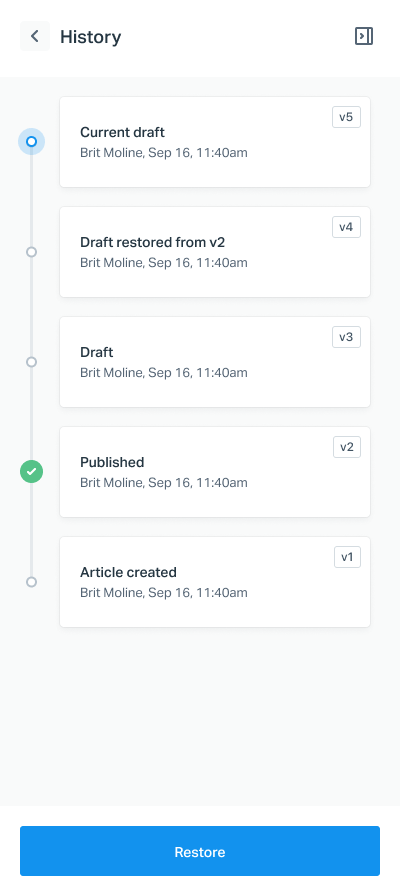A detailed screenshot of a mobile phone interface is displayed. The top part of the image has a white background with black text. On the left, there's a back arrow labeled "History," and on the right, there's a three-dimensional square shape with an arrow pointing to the right.

Below this header, on a gray background, there are five white rectangles vertically aligned. The details of each rectangle are as follows:

1. The first rectangle features a blue circle adjacent to black text that reads "Currency Draft, Brit Monley, September 16th, 11:40 A.M." In the upper-right corner, it is labeled "V5."
2. The second rectangle shows a gray circle next to the text "Draft restored from V2, Brit Monley, September 16th, 11:40, V3," further marked with "V4."
3. The third rectangle contains a circle labeled "Draft, Brit Monley, September 16th, 11:40, V3."
4. The fourth rectangle has a green circle with a white checkmark, indicating "Published, Brit Monley, September 16th, 11:40, V2."
5. The fifth rectangle, again with a gray circle, reads "Article created, Brit Monley, September 16th, 11:40, V1."

At the very bottom, there is a large blue rectangle with the word "Restore" printed in white. It suggests functionality related to restoring a previous version.